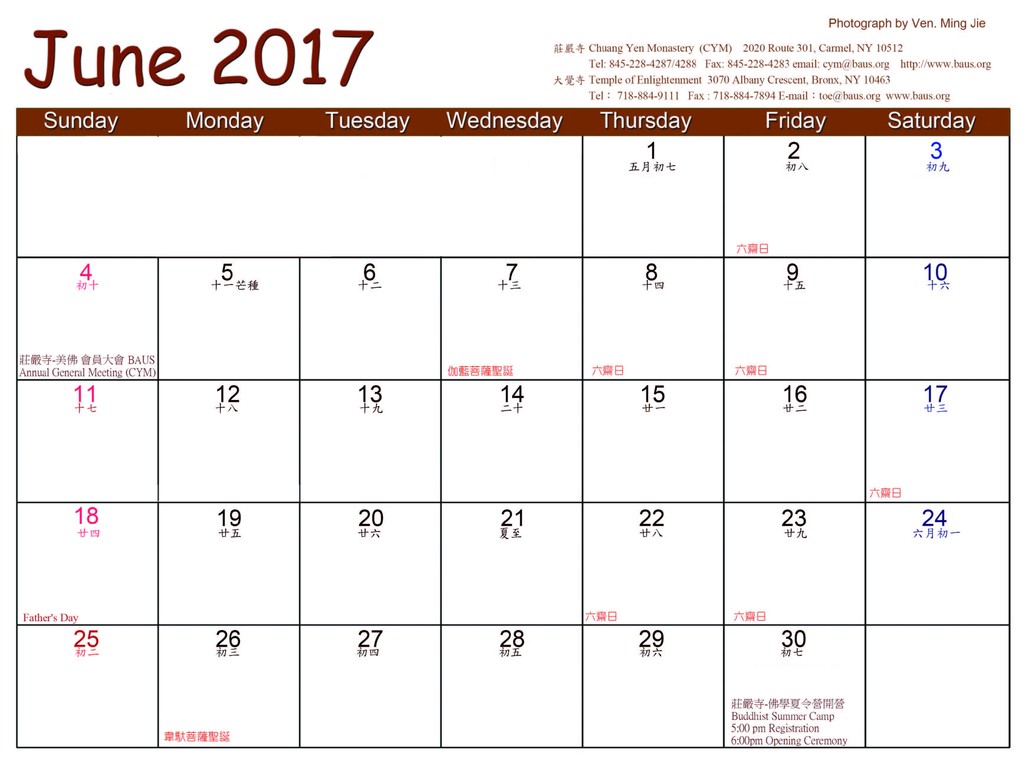This image depicts a digital calendar for June 2017. The background is white, with "June 2017" prominently displayed in bold brown letters in the upper left corner. Below this, there is a blue horizontal strip, featuring the days of the week—Sunday, Monday, Tuesday, Wednesday, Thursday, Friday, and Saturday—written in white text. The main calendar area consists of several rectangles and squares representing each day of the month, numbered from 1 to 30. Each date square contains text written in an Asian language, likely Japanese or Chinese. In the upper right corner, there is additional small text that reads: "Photographed by Ven Ming-Chi." Beneath this, there is more information in Chinese characters, followed by "Chuang Yen Monastery, CYM, 2020 Route 301, Carmel, New York, 10512," and "Temple of Enlightenment, 3070 Albany Crescent, Bronx, NY, 10463." This detailed composition provides a clear and informative view of the calendar.